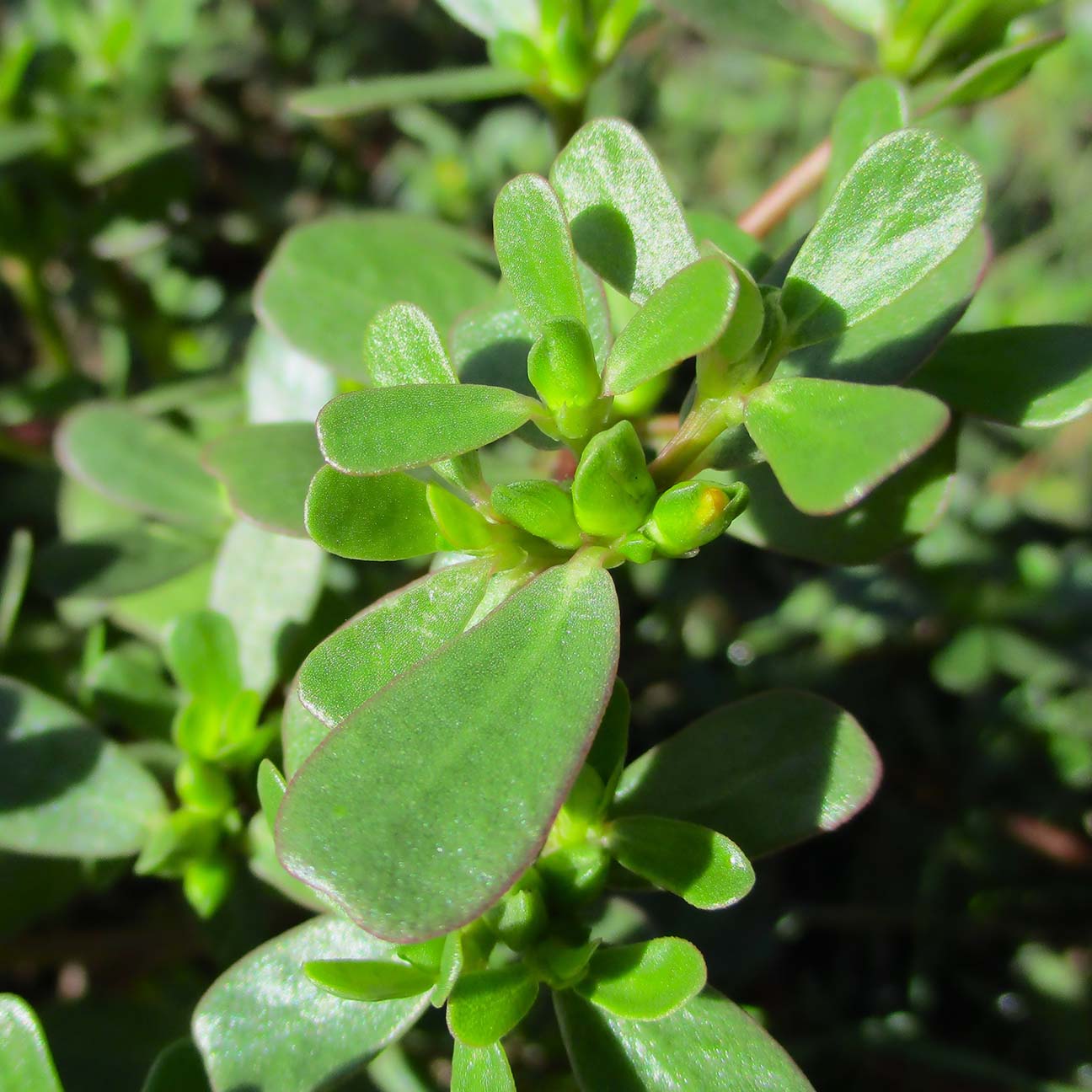This photograph is a detailed close-up of a succulent plant, showcasing its vibrant, green leaves. The leaves are broad, uniform, and have a striking tinge of purple on their edges, which is particularly visible on the larger leaves. The image captures the plant's new growth emerging from the center, emphasizing the fresh, tender leaves. While the central plant is in sharp focus, the background features an array of out-of-focus greenery, adding depth to the composition. The succulent's slightly thick, juicy leaves suggest they might store some substance inside, enhancing their lush appearance. Overall, the vivid green and subtle purple hues create a captivating and lively image.